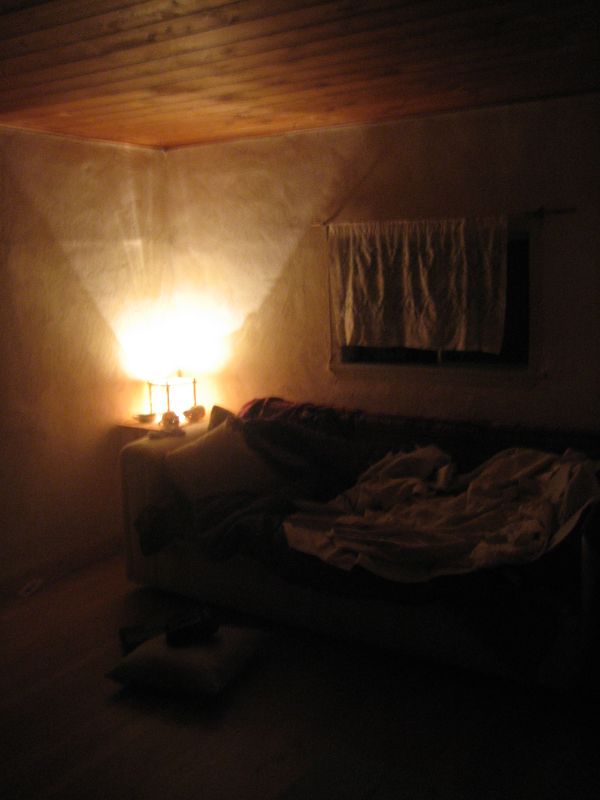This indoor setting, captured in a photographic style, resembles a dark, eerie living space. The dominant feature is a tunnel-like structure, stretching from the foreground's deep blackness—occupying around two-thirds of the image—toward a glowing bright orange light at the end. Adding to this unsettling ambiance, the straight, man-made walls guide the viewer’s gaze down the tunnel. On these stucco walls, several gray curtains or panels are visible, lending the scene an additional layer of mystery. 

In front of the distant orange light, a trio of box-like shapes with protruding poles stand out as shadowy silhouettes. Their shapes cast reflections, with the light scattering off the tunnel's walls and ceiling, enhancing the scene's suspenseful atmosphere. Despite some elements suggesting a typical room—a sofa draped with light and dark blankets, a cushion on the floor, and potentially a small window covered by a curtain—the overall darkness conceals specific details, leaving much to the imagination. This composition blurs the line between a living room and a passageway, evoking the feeling of a horror movie set, with a sense of foreboding amplified by the strong contrast of light and shadow.